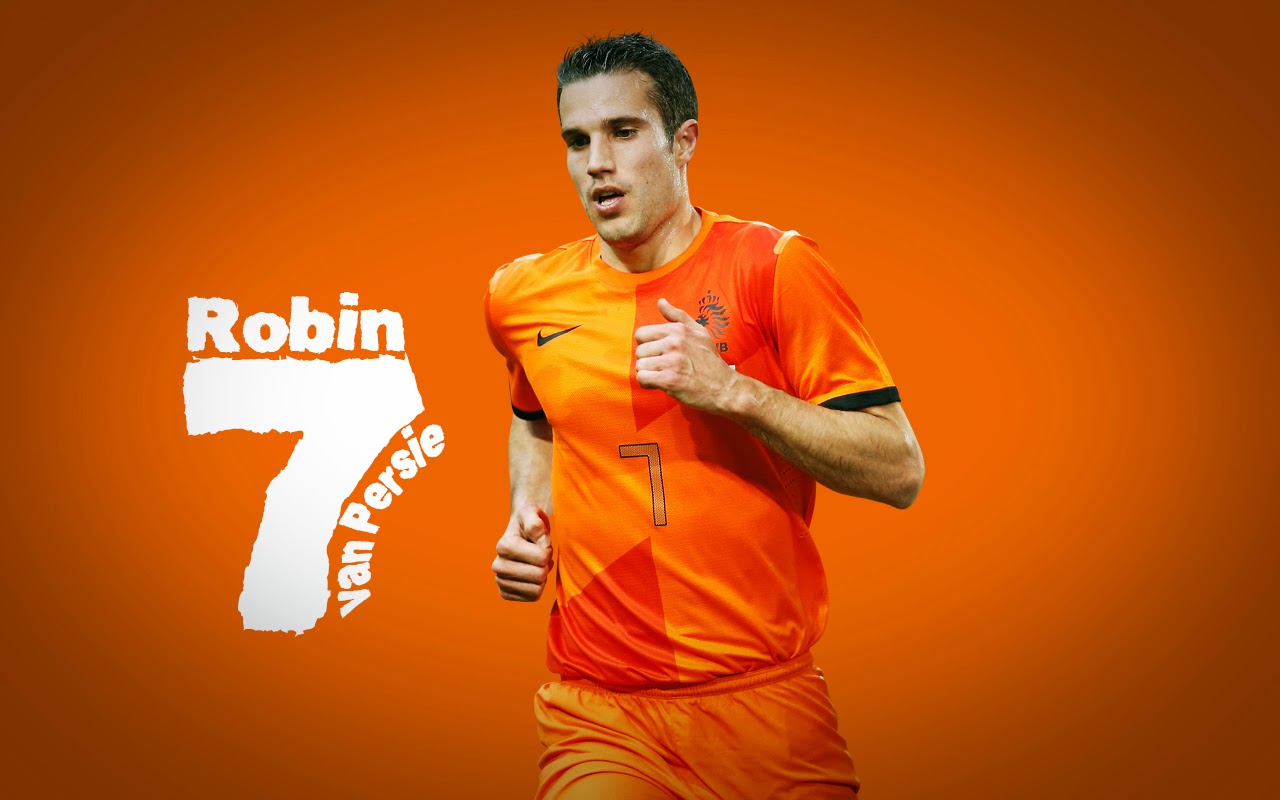The image features a soccer player in mid-run, positioned centrally against an orange background that gradually darkens towards the edges. The athlete, identified as Robin Van Persie through text on the left side of the image, has short brunette hair and an olive complexion, with sweat visible on his brow. He is wearing a predominantly orange jersey that includes dark orange triangular designs emerging from the shoulder and lower part of the shirt. The jersey also features a black Nike swoosh on the top left and a large white number 7 prominently displayed in the center. The sleeves of the jersey have black collars, and he is also wearing matching orange shorts. The text "Robin" appears above the number 7, while "Van Persie" curves around the lower part of the 7.